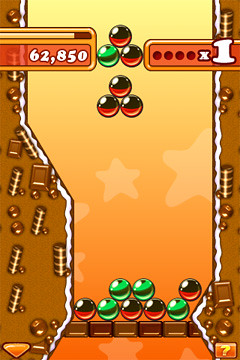A detailed and cleanly formulated descriptive caption for the image might be:

"The screenshot is from a mobile game featuring a vertically aligned, rectangular interface. The scene captures a section where a hole with a soil wall is visible. This soil wall contains a few embedded items and gives way to a serene, evening sky backdrop adorned with star-shaped clouds. In the center of the screen, black and green marbles are being dropped onto a rope. These marbles land on a blocked-off path, preventing others from falling. On the left side of the screen, there are two visible sections: one displays various numerical types, while the other shows the current score."